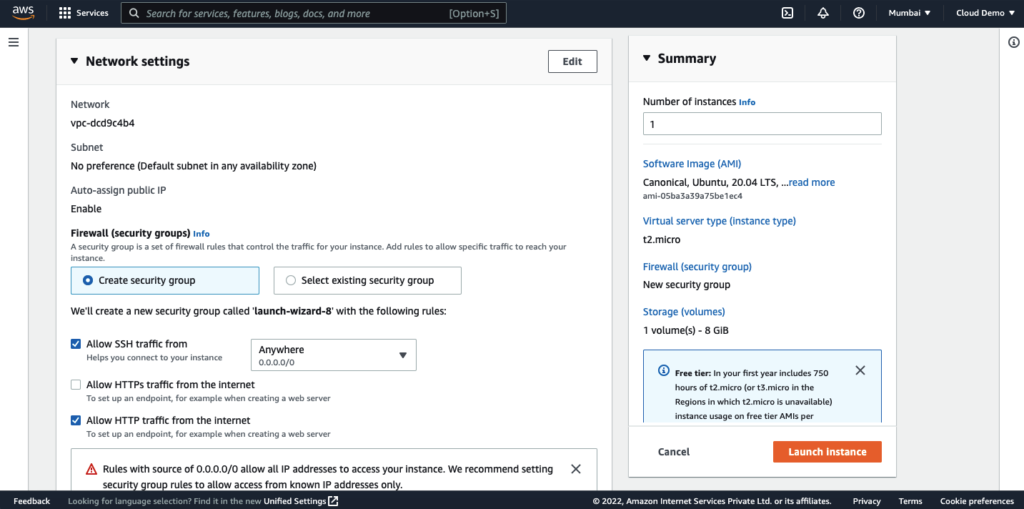The provided image is a detailed screenshot of an AWS interface, prominently displayed in the upper left corner. Below the header that reads "AWS," there is a "services" button. Adjacent to this, a search bar is labeled with the placeholder text "search for services, features, blogs, docs, and more." Continuing to the far right, there are three icons: the first one is indistinct, the second resembles an upward-pointing arrow, and the third is a circular icon with a question mark inside. Additionally, there are two drop-down menu buttons; the first is illegible, but the second appears to be labeled "cloud demo."

Beneath this header section, on the left side of the image, there is a heading that reads "network settings." Below this, a network address is displayed, followed by the text "subnet," which is set to "no preference." Further down, a section titled "firewall security groups" indicates that the selected option is "create security group," specifying that a new security group named "launch wizard 8" will be created with specified rules. This section includes several checkbox options.

On the right side of this interface, there is a "summary" section. This includes a "number of instances" heading, with a text box underneath that contains the numeral "1."